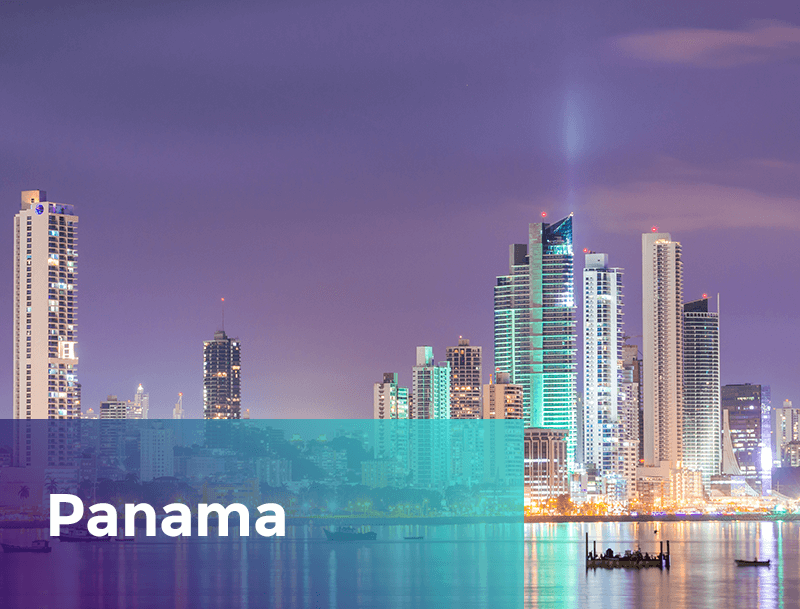The image portrays a mesmerizing nightscape across a river, showcasing the skyline of Panama City. Dominating the scene are numerous high-rise buildings, their illuminated facades casting vibrant reflections in the water below. The palette of the city lights ranges from purple to blue, creating a stunning visual contrast against the night sky. At the bottom left corner, the name "Panama" is prominently displayed, anchoring the viewer's location. Among the skyline, one tower stands out with a powerful searchlight beaming upwards, piercing the darkness. In the foreground, a few boats drift lazily on the river, subtly adding to the tranquil yet dynamic ambiance of the scene.